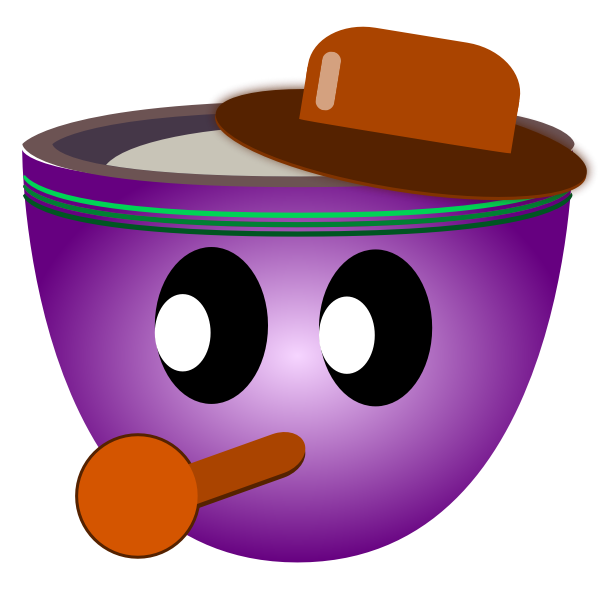The image features a detailed cartoon rendering of a tall, handle-less purple teacup or bowl, gradually changing to a lighter purple towards its center. It has two large oval eyes with smaller white ovals serving as pupils, both eyes gazing towards the left. Where the nose or mouth would typically be, there's a protruding stem ending in a ball-like shape, resembling a pipe. Adorning the top right of the bowl is a wide-brimmed hat in a mix of brown and dark brown hues. The hat addition gives the cartoon character a whimsical, party-like appearance. Additionally, the bowl or teacup seems to contain a gray liquid. The upper edge of the bowl has a green trim, adding to the quirky and colorful design.